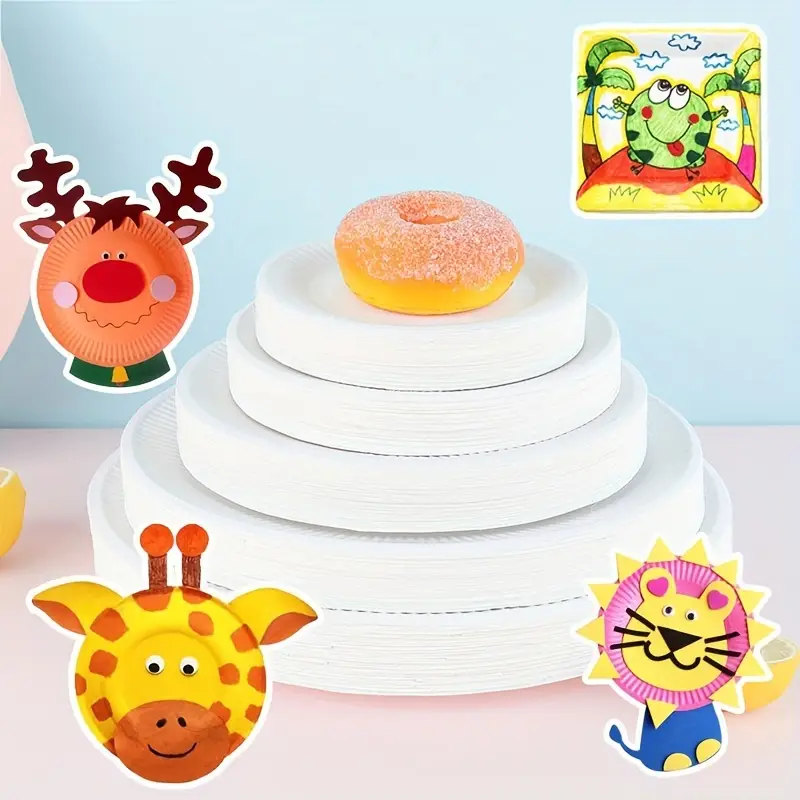This vibrant color photograph showcases a range of creative paper plate crafts against a light blue background, set atop a pink tablecloth. Dominating the center is a striking five-tiered stack of white paper plates, arranged from largest at the bottom to smallest at the top, topped with a bright pink sugar-coated donut.

Surrounding this central stack are four playful paper plate designs, each occupying a corner of the image. In the top left corner, a reindeer crafted from paper plates stands out with antlers, ears, a green sweater, and a prominent red nose. The top right corner features a square paper plate decorated with a child-like crayon drawing of a frog in vibrant colors. The bottom left showcases a cheerful lion created from paper plates in bright hues. Finally, the bottom right displays a whimsical giraffe, complete with googly eyes, ears, and horns, also constructed from a paper plate.